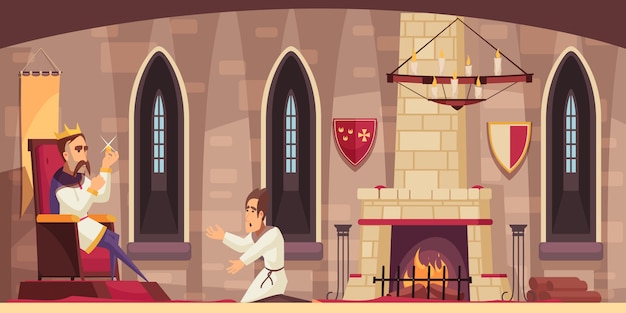The detailed 2D illustration, crafted in a flat cell animation style, depicts an interior palace setting, dominated by a rich red and gold color palette. At the center, a bearded king, adorned in a gold crown and a royal ensemble featuring purple and gold accents, sits on a throne with a dark red cushion and brown base. The king holds a shiny object, likely a gemstone or a diamond, and scrutinizes it with a neutral expression. In front of him, a distressed peasant or servant, dressed in a coarse white robe cinched with a rope, kneels and appears to be pleading.

The scene is illuminated by an iron chandelier with lit candles, casting a warm glow that complements the flickering light from the nearby fireplace, which has a gold chimney. The walls are adorned with red and gold banners and shields, possibly coats of arms, and the background features narrow oval windows with glass panes. The overall composition of the illustration evokes a dramatic moment of supplication within a richly decorated regal chamber.